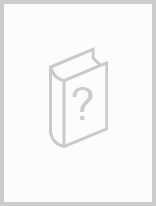The image is a black and white pamphlet-style collage, likely a memorial, featuring three photographs. The top half showcases two pictures: on the left, a very young boy with dark hair, resting his left cheek on his hand and wearing a white shirt, and on the right, a teenager or young man, possibly the same individual grown up, with dark hair and a black jacket with a collar. The bottom half of the pamphlet displays a single photograph of an older man wearing a fedora with a black band and a black trench coat. He is positioned with his right hand on the brim of the hat, partially obscuring his face. A bar of light purple runs horizontally across the middle of the pamphlet, featuring the dark purple text "Juan Jose Girola" above which the word "Memorias" is written in purple. At the bottom right of this purple bar, the words "Ediciones El Milagro Conocota" are printed in pink.